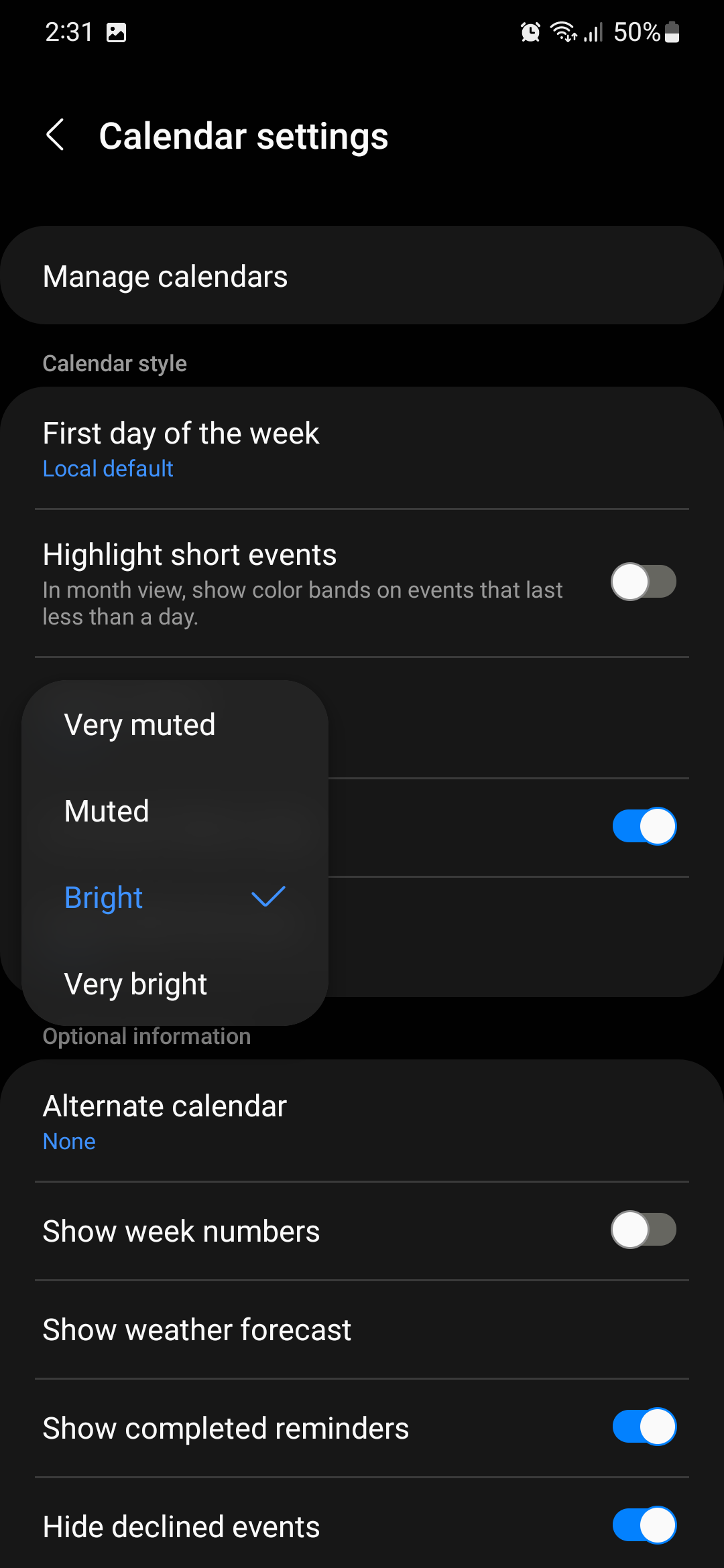Here is the detailed caption:

"The image depicts a smartphone screen with a predominantly black background. At the top left, '2:31' is displayed in white, indicating the time. To the right of the time, there is a small white image icon. Further right, an alarm clock symbol, a Wi-Fi symbol with down and up arrows, a set of data signal bars, and a 50% battery icon are visible. The battery icon is half full.

Below this bar, there is a thin white arrowhead pointing to the left, followed by the bold text 'Calendar Settings.' Below this text, a dark gray oval contains the white text 'Manage calendars.' The background transitions back to black, and on the left side, in very small gray font, 'Calendar style' is written.

Underneath this text, there is a rounded rectangular section with a dark gray background. In white letters, it reads 'First day of the week,' and beneath that, in small blue lettering, it says 'Local default.' A long gray line serves as a divider below this.

Further down, the text 'Highlight short events' appears in white. In smaller light gray lettering beneath that, it says 'In month view, show color bands on events that last less than a day.' To the right of this text, there is a toggle option. It is turned off, indicated by a circular white icon positioned to the left within a gray oval area.

Towards the left of the screen, a notification or extra menu has popped up. The options listed are 'Very muted,' 'Muted,' 'Bright,' and 'Very bright.' All the options are in white, except for 'Bright,' which is highlighted in blue with a blue checkmark to the right."